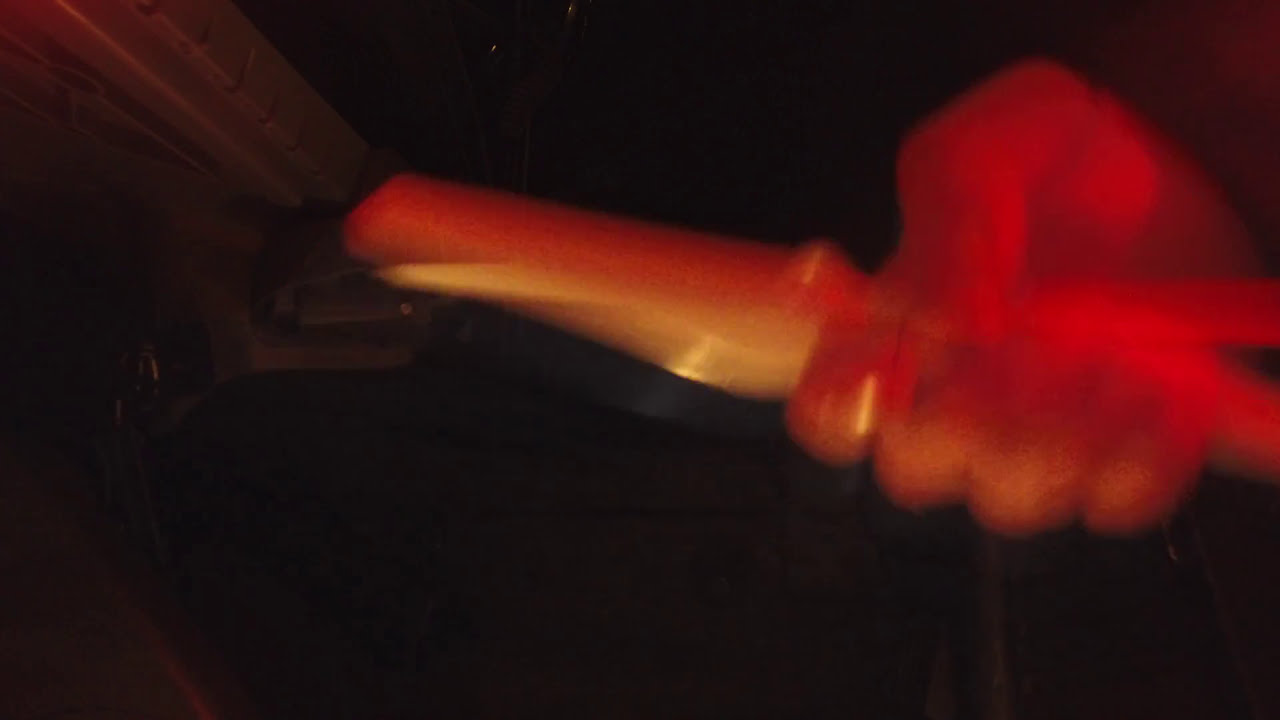In this horizontal rectangular photograph taken at night, the image is predominantly dark, with a striking red and orange area on the right side extending past the middle. This area appears to be a building illuminated by lights, giving an impression reminiscent of flames due to the vivid colors, though no actual flames are visible. The building features a canopy-type structure on top and seems to be constructed of concrete, bathed in reddish-orange hues. Around the bottom of the building, lighter colors, predominantly yellow with a scalloped pattern, suggest the presence of pillars or architectural details.

Emerging from the top right of the image is a hand, tinted orange by the surrounding light, holding two indistinct, possibly metallic objects. The hand and the objects are very blurry, exhibiting motion blur because the hand was moving when the picture was taken. The background behind the hand is dark, with dim grayish hues, hinting at an indoor setting but offering no clear details due to the poor visibility and low light conditions.